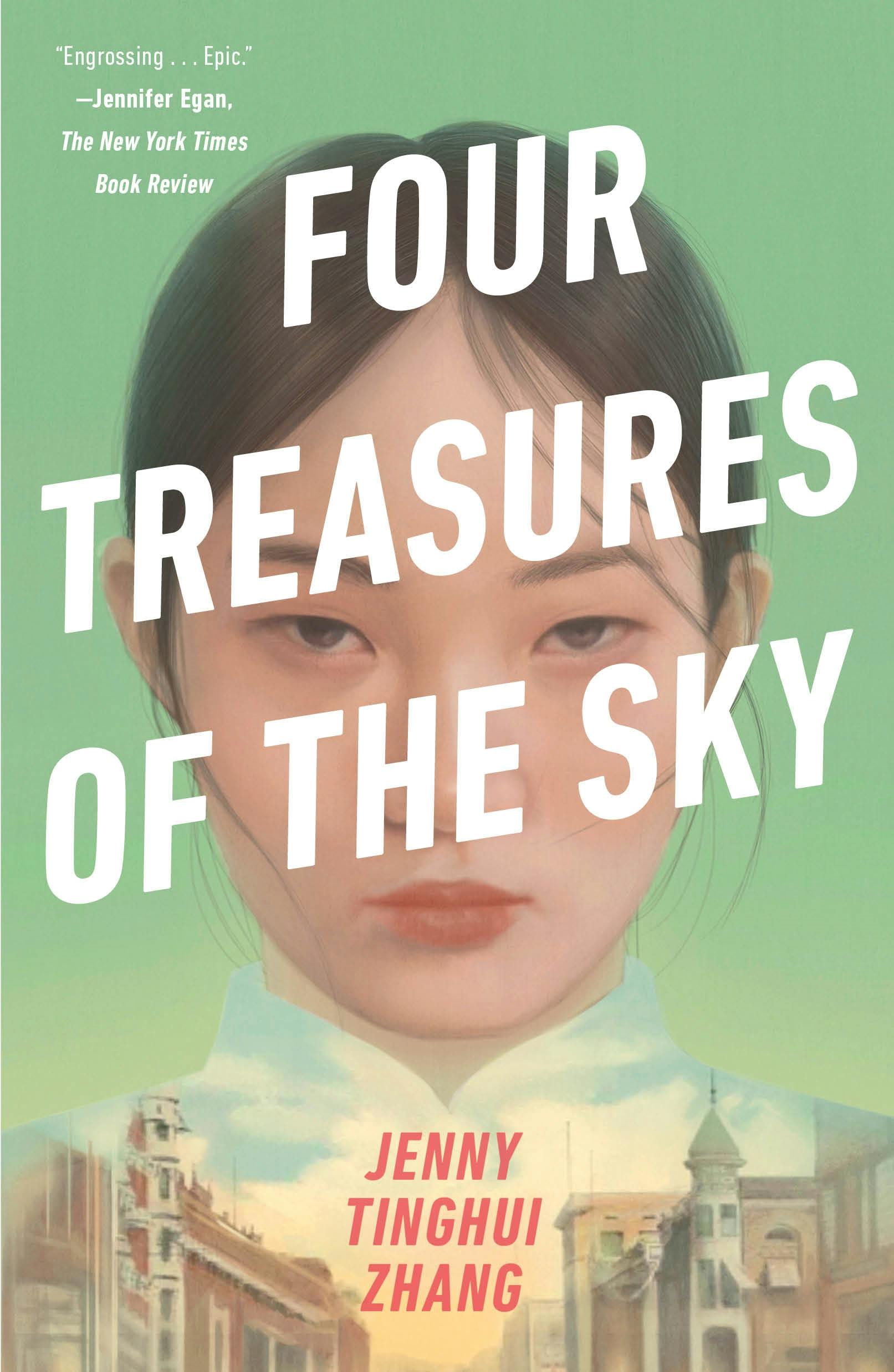The cover of the book features a striking and detailed illustration set against a light green background that deepens in shade towards the top. Dominating the center is the head of a young Asian girl with black hair parted in the middle and tied back, her expression stern and her face egg-shaped. Across her face, in large, bold white capital letters, is the book's title: "FOUR TREASURES OF THE SKY." Below this title, beneath the girl's chin, is an ethereal depiction where her white-collared shirt merges seamlessly into a sky filled with blue clouds, and two brown buildings emerge on either side, creating a cityscape. In red letters just below, the author's name is elegantly displayed: "Jenny Tinghui Zhang." At the top left corner of the cover, a review from Jennifer Egan of The New York Times Book Review calls the book "Engrossing... Epic."